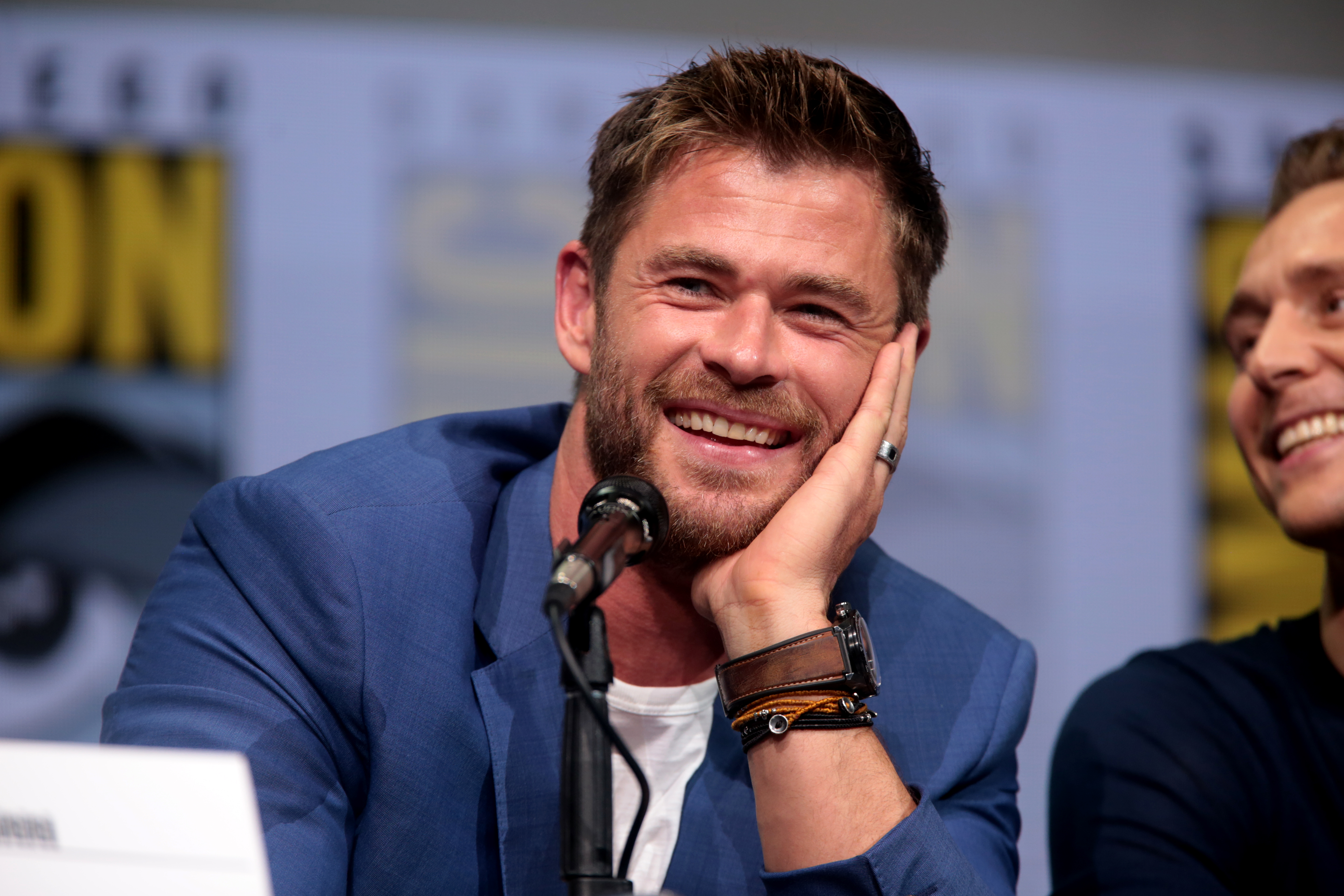This is a detailed photo shot at a Comic-Con event, identifiable by the Comic-Con logo on a white banner in the background. The focal point is a muscular gentleman with short, dark brown hair styled up in the front, a short beard, and a leather-banded watch along with bracelets. He is wearing a blue cloth suit jacket over a white t-shirt and is smiling warmly while holding his head with his left hand. Adding to his look, he also wears a ring. Next to him is a skinnier man in a dark shirt, smiling and laughing while holding a microphone, suggesting he might be mid-conversation or conducting an interview. The photo captures the lively, engaging atmosphere typically found at such conventions, with the backdrop featuring indistinct text and colors ranging from dark blue, royal blue, brown, tan, silver, black, mustard yellow, white, and gray. Both men are clearly enjoying their time, indicative of the indoor Comic-Con setting, although the exact time of day remains unclear.